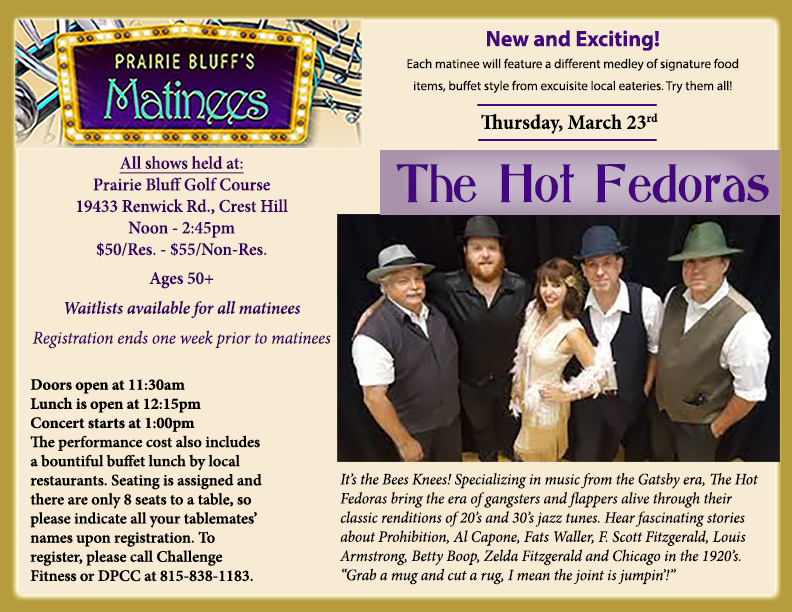This image is a promotional ad for the Prairie Bluffs Matinees, prominently displaying a marquee at the top left reading "Prairie Bluffs Matinees." The event is hosted at Prairie Bluffs Golf Course, located at 19433 Renwick Road, Crest Hill. The ad details that shows are priced at $50 for reservations and $55 for non-reservations, catering to an audience aged 50 and above. A waitlist is available, with registration closing one week prior to the matinees. Doors open at 11:30 a.m., lunch begins at 12:15 p.m., and the concert starts at 1 p.m., concluding at 2:45 p.m. The show on Thursday, March 23rd features The Hot Fedoras, a music group consisting of four men and one woman, positioned centrally in the photograph. Additionally, the ad highlights that each matinee will offer a unique assortment of signature dishes from local eateries. The overall design has the appearance of a yellow-card-style poster fit for online and print promotion.